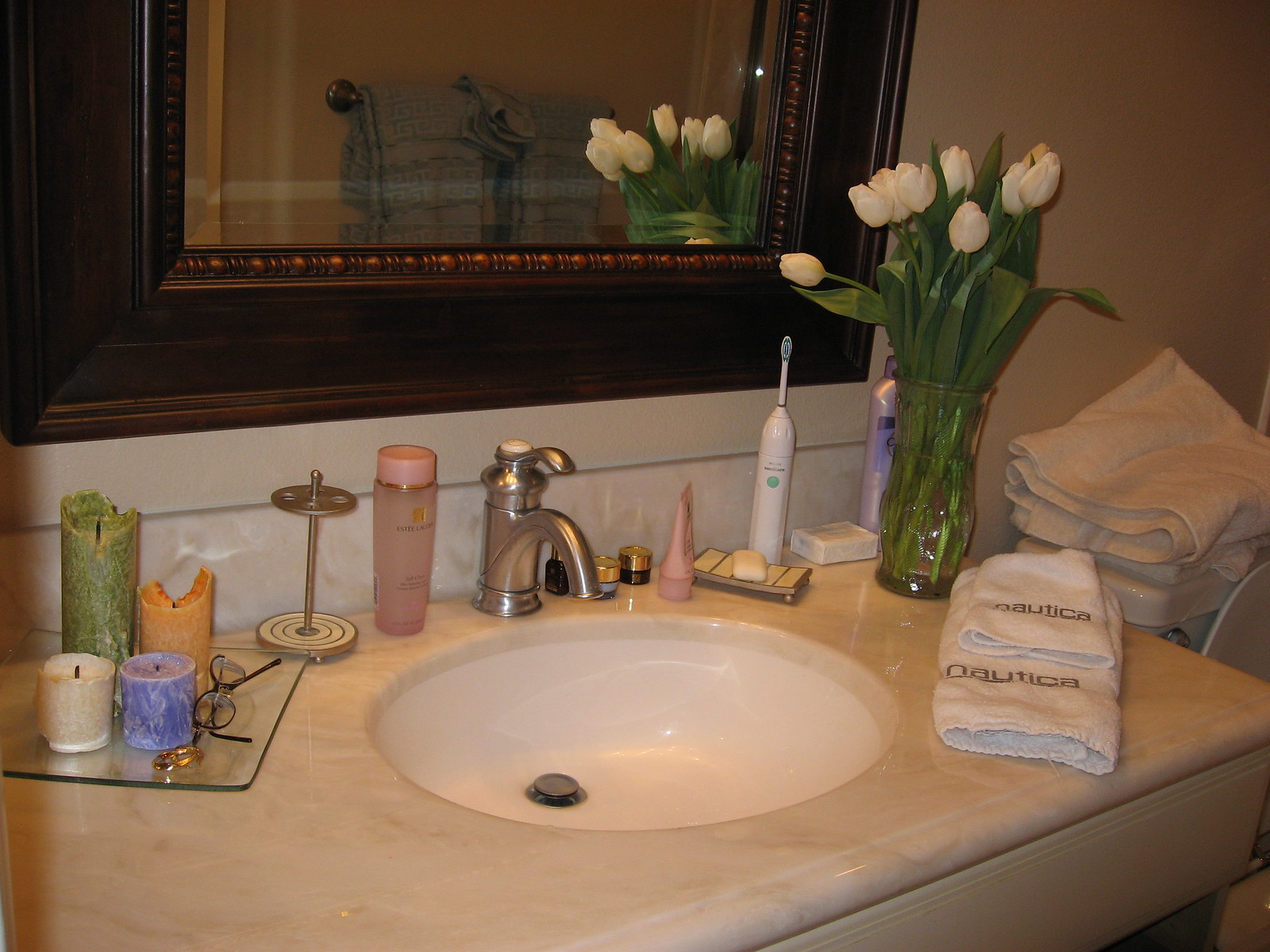The image depicts a luxurious and exquisitely decorated bathroom. The centerpiece is a stunning vanity with an integrated sink, seamlessly blending into the countertop without a lip. The elegant design is complemented by a sleek single-spout faucet.

On the vanity, a glass tray holds an assortment of vibrant candles in hues of green, orange, purple, bluish-purple, and cream, all in varying heights. Nearby, a toothbrush holder stands empty, and a bottle of toner, enclosed in a pink container with a matching cap, adds a splash of color. Adjacent to the faucet, small jars and a pink tube, presumably containing lotion, are meticulously arranged alongside a soap dish holding an unused bar of soap. An electric toothbrush is positioned behind this arrangement.

A touch of nature is introduced by a clear vase filled with white tulips, their stems submerged in water, adding a refreshing and tranquil element to the space. Next to the vase, a bottle believed to be body lotion is discreetly placed.

Two white towels bearing the Nautica logo rest neatly on the right side of the countertop. Additionally, more white towels are thoughtfully stacked on top of the toilet, providing both practicality and elegance.

The focal point of the bathroom is a striking mirror with a thick, wood frame adorned with an intricate braided design on the inner edge. The reflection in the mirror reveals a set of green towels hanging across from the sink, completing the harmonious and sophisticated aesthetic of the bathroom.